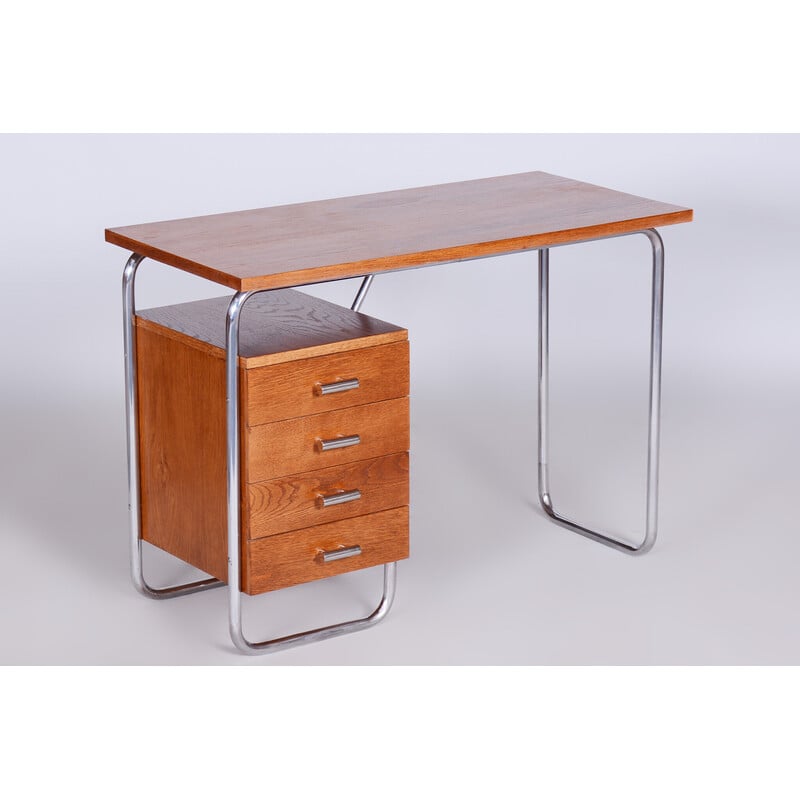This is a very simple, horizontally rectangular, full-color photograph taken indoors with artificial light. The image features a small wooden desk set against a stark white floor, with no other colors or objects visible in the background. A gray shadow is cast on the floor, indicating artificial lighting in the room. The desk has a polished rectangular wooden top, and it is supported on the right side by simple shiny silver metal legs that form a rectangular frame. On the left side, the support structure extends into a four-drawer cabinet, wrapped in the same shiny silver material holding the table. The drawers themselves are made of polished hardwood, matching the desk's top. Overall, the desk is meticulously clean and free of clutter, emphasizing its minimalist, sleek design.